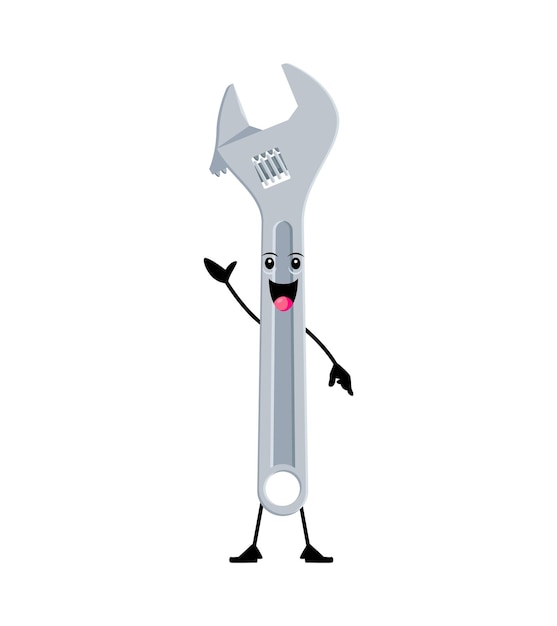This is a detailed vector image of a cartoon-stylized adjustable wrench depicted with anthropomorphic features against a plain white background. The light gray wrench stands upright, facing the viewer, and exhibits human-like characteristics. At the center of the wrench body, there's a smiling face with expressive black eyes and eyebrows, an open mouth, and a bright pink tongue sticking out. The wrench has two arms; the right arm is waving enthusiastically at the camera, while the left arm points downward. Additionally, it stands on two legs donning black shoes. The wrench is partly open at the top, revealing detailed mechanical structures, including a rectangular latching mechanism and a small circular ring towards the bottom. The overall design incorporates both light and dark gray shades, adding depth and dimension to the whimsical character.